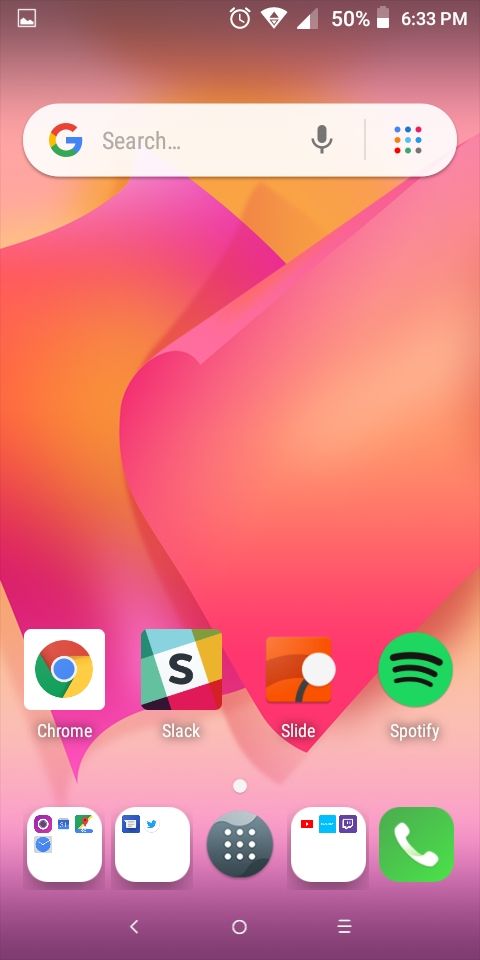The image depicts a cell phone screen with multiple icons and features. In the top right corner, icons for an alarm clock, wireless connection, cellular connection, and battery status are visible, alongside the indicators showing "50%" battery and the time "6:33 PM". The background consists of a swirled and variegated pattern in shades of pink and orange.

At the top of the screen, a search bar adorned with the Google logo on the left side reads "Search..." and includes a microphone icon for voice search. Below this search bar, four prominent app icons are aligned horizontally: 

1. The first icon is a square with the Google Chrome logo and the label "Chrome" underneath.
2. The second icon is a square with a colorful design and an 'S' in the middle, labeled "Slack".
3. The third icon is a square with an orange background and a white circle inside, labeled "Slide".
4. The fourth icon is a green circle featuring three black horizontal lines, labeled "Spotify".

At the bottom of the screen, another set of icons is displayed, featuring four squares and a central circle:

1. The first square contains several smaller icons, one of which is a clock.
2. The second square, slightly to the right, includes two icons, one of which is the Twitter symbol.
3. The central circle is predominantly black with nine small white dots arranged within it.
4. The third square, appearing as a rounded rectangle, contains three logos including what seems to be the YouTube logo.
5. The final icon is a green square with a white phone symbol, indicating it’s for phone calls.

Each detail contributes to a comprehensive snapshot of the cell phone screen interface.